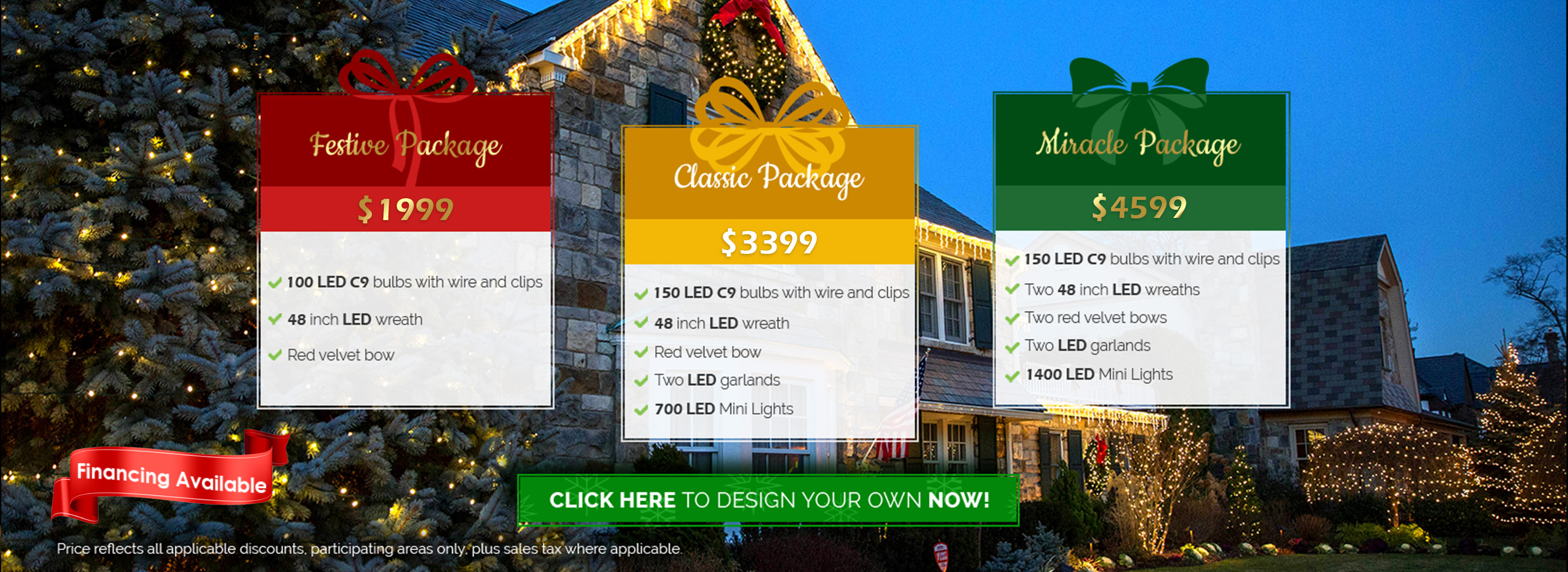The image, taken at dusk, depicts a picturesque suburban neighborhood adorned with festive Christmas decorations. The sky is tinged with a soft bluish hue, providing a serene backdrop for the illuminated houses. The homes are brilliantly lit with an array of Christmas lights, wrapping around not only the structures but also the trees in the front yards. 

Prominently featured is a house with an A-frame roof, adorned with a giant wreath where the roof's sides converge. The wreath is beautifully illuminated and accented with red fabric, adding a notable focal point to the festive display.

In the foreground, there are three festive boxes, each with distinctive colors and text. The box on the left is red and labeled "Festive Package $1,999," with additional, smaller text that is unreadable. The center box is gold, marked "Classic Package $3,399," also featuring smaller unreadable text. The box on the right is green, bearing the inscription "Miracle Package $4,599," with an additional prompt beneath it, stating "Click here to design your own now."

This enchanting scene blends the warmth of holiday spirit with the serenity of an impending winter's night, punctuated by inviting offers for customizable holiday decorations.